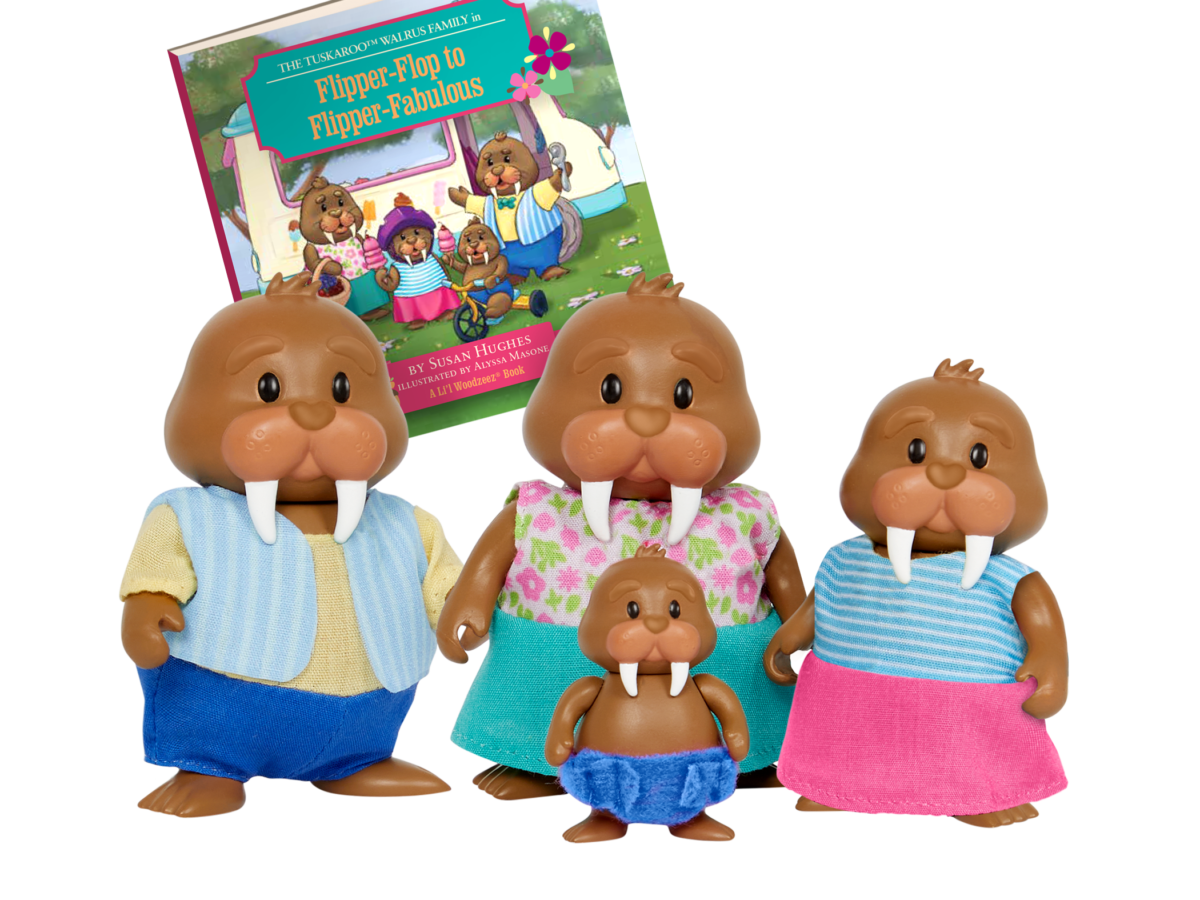This image features a colorful children's book titled "The Tuscaroo Walrus Family in Flipper Flop to Flipper Fabulous" by Susan Hughes, illustrated by Alyssa Messone, with the Lil Wood Z's branding. The square-shaped book depicts a whimsical adventure of a walrus family including a father, mother, daughter, and baby, illustrated in front of what appears to be a white family van. In the foreground, there are four detailed figurines that match the characters on the book cover. The father walrus is dressed in a blue vest, blue shorts, and a yellow shirt, while the mother wears a blue skirt and a flowered top. The daughter sports a pink skirt and a blue striped top, and the baby walrus is in a blue, jean-like diaper. Each figurine is brown with distinctive white tusks, perfectly mirroring their literary counterparts and bringing the adventurous family to life.